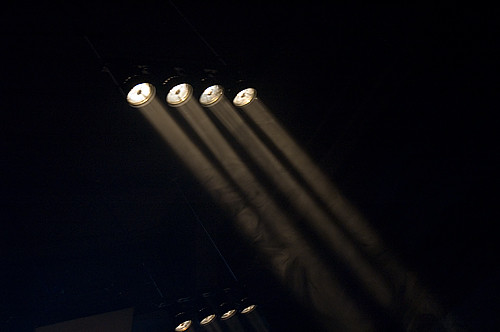The photograph captures a dimly lit, indoor scene reminiscent of a theater or concert hall. The background is entirely black, emphasizing the central focus of the image: four spotlights aligned in a row, suspended overhead. These spotlights, with their cylindrical steel bodies and shiny silver caps, emit a bright white light, casting beams that playfully interact with the surrounding darkness. In the glow of these lights, wisps of dust or smoke can be discerned, adding a textured, almost ethereal quality to the scene. Below these spotlights, near the bottom center-left of the image, there appears to be another set of four lights, positioned at a slight incline. These could be either footlights on a stage or mirrored reflections of the overhead spotlights, casting a subtle glow without the intensity of the primary lights above. The photograph's blurry focus and slight haze contribute to its enigmatic and atmospheric nature.